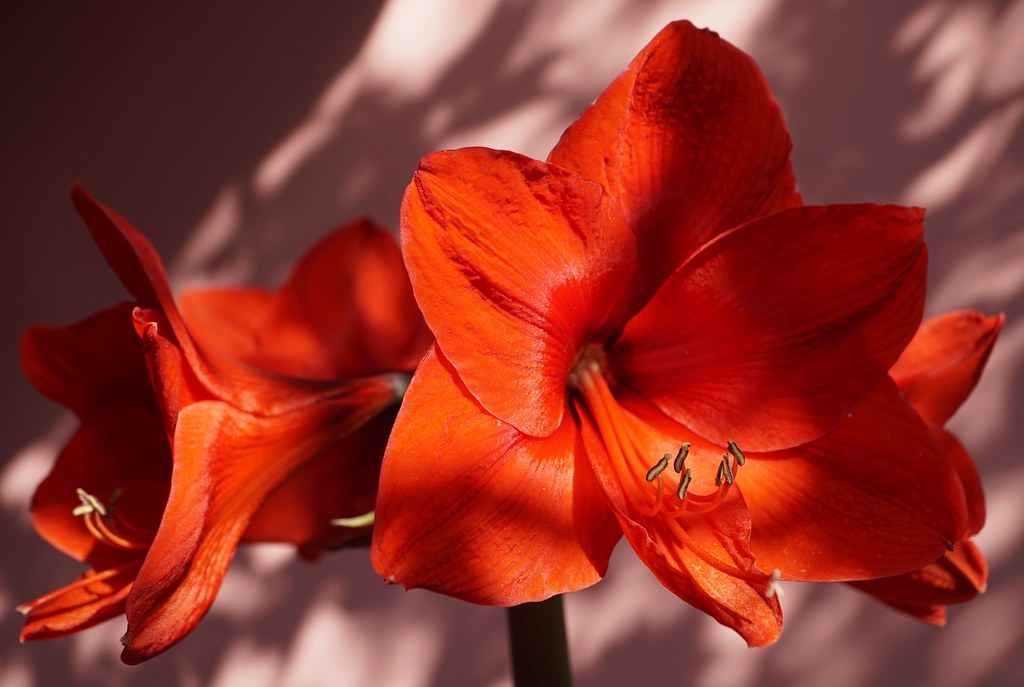This close-up image depicts two vibrant flowers standing out against a stark white background, which is accentuated by dark shadows resembling branches. The flowers, primarily deep red with hints of orange and yellow, display their striking details prominently. Both blooms appear to be part of the same plant, sharing a thick green stem that extends downwards from the central area of the frame. The petals of these flowers are oval with pointed tips, and each flower has long, thin red filaments emerging from its center, ending in small black seed-like structures. The flower on the right angles slightly to the right, revealing its interior with six distinguishable filaments, while the one on the left, oriented to the left, offers a more shadowed view. The interplay of light and shadow suggests an indoor setting, possibly near a window, creating a dynamic contrast on the wall and the flowers.